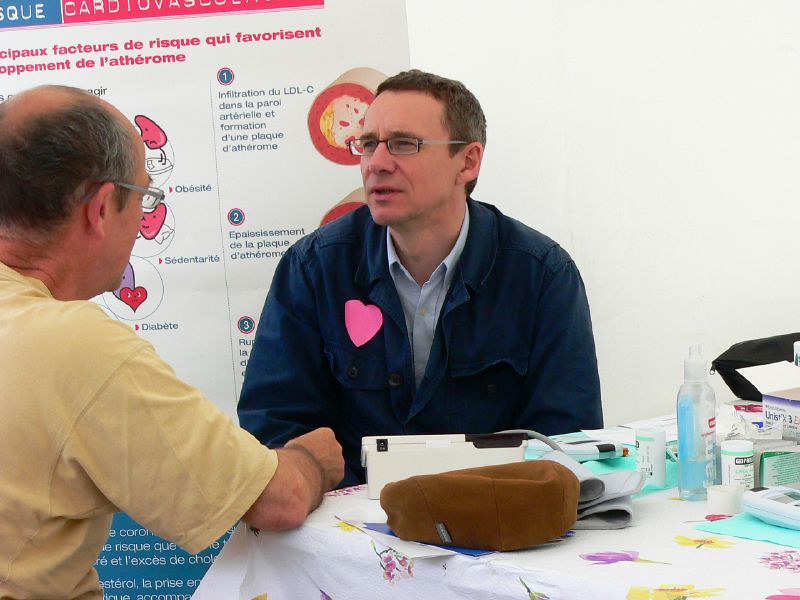The photograph, captured in a landscape layout, prominently features two Caucasian men engaged in conversation at a table adorned with a multicolored tablecloth and a variety of medical items, including CPR equipment and breathing apparatuses. The man at the center of the image, likely in his mid-fifties, is seated and visible from the waist up. He wears a navy jacket with a pink heart emblem and a blue button-down collared shirt underneath. His brownish-gray hair, glasses, and thoughtful expression complement his attire. To the left corner of the image stands the second man, viewed from behind. He sports a light yellow short-sleeved shirt, glasses, and balding brown hair. This man appears to be elderly, possibly in his mid-sixties, and is deeply engaged in conversation with the seated man, who might be a medical professional offering guidance. The backdrop features a white wall adorned with red, blue, and white banners displaying circulatory diagrams and healthcare-related text, hinting at a health or wellness event focused on elderly care and heart health.